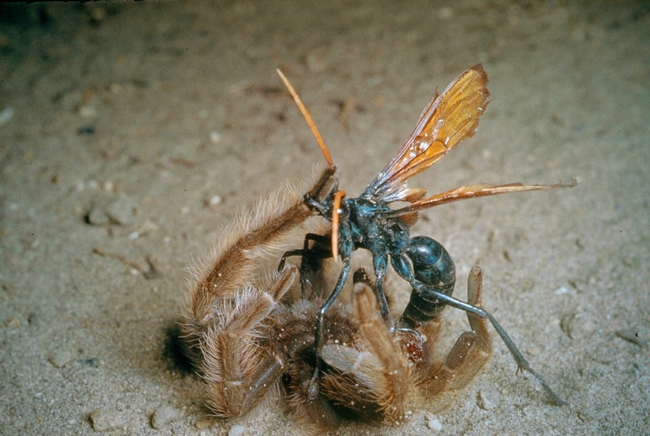This is a detailed, zoomed-in photograph capturing a dramatic scene between a spider and a predatory wasp in an outdoor setting, possibly during the evening. The backdrop is dirt, illuminated by a light source coming from behind the camera to the right. A black tarantula-like spider, distinguishable by its fur-like hairy legs, lies on its back with limbs raised, suggesting it might be dead or incapacitated. Straddling the spider is a black wasp with distinctive amber-colored wings that are veined darkly and light tan antennae, hinting that this is a tarantula hawk. The wasp grips part of the spider, showcasing the intense interaction. The image highlights two well-defined wings of the wasp and the black, segmented body of the insect, emphasizing the powerful stillness of the spider and the alertness of its captor.